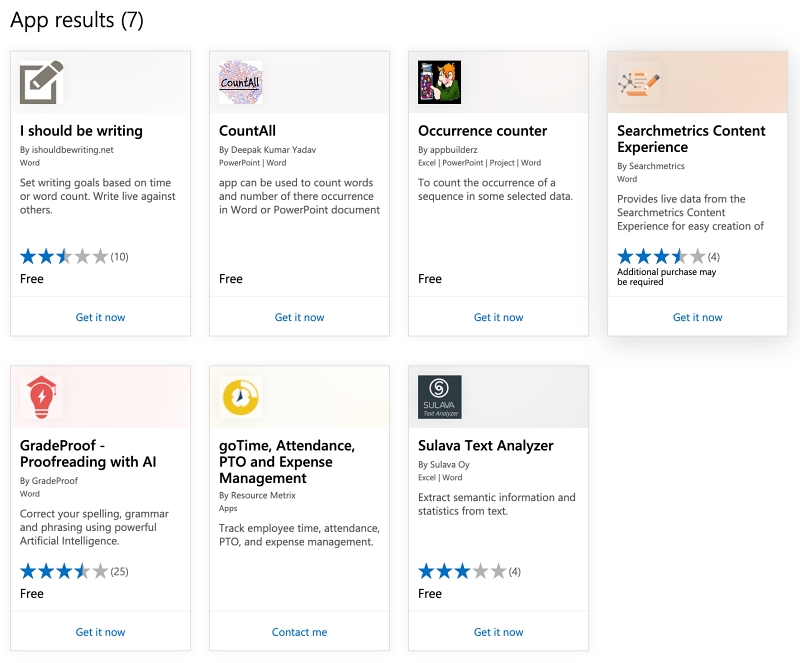The image displays a compilation of app results, shown in a series of rectangular sections. The first rectangle highlights an app titled "I Should Be Writing," which focuses on helping users set writing goals based on either time or word count. It also includes a feature to write live against others. This app has received 10 ratings, averaging 2.5 out of 5 stars.

The second rectangle presents the "Count All App," useful for counting words and the occurrences of specified terms in Word or PowerPoint documents. Another feature in this app is the "Occurrence Counter," which counts sequences in selected data.

Next, the "Searchmetrics Content Experience" app is shown, which offers live data from the Searchmetrics Content Experience to simplify content creation. This app has 4 ratings, averaging 3.5 out of 5 stars.

Following that is "Great Proofreading with AI," which utilizes artificial intelligence to correct spelling, grammar, and phrasing. This app has 25 ratings, averaging 3.5 out of 5 stars.

Lastly, the "Go Time Attendance, PTO, and Expense Management" app is listed, which helps users track employee time attendance, PTO, and expense management. There is also a mention of the "Sulava Text Analyzer," spelled "S-U-L-A-V-A," though the detailed information or ratings for this app are not provided in the text.